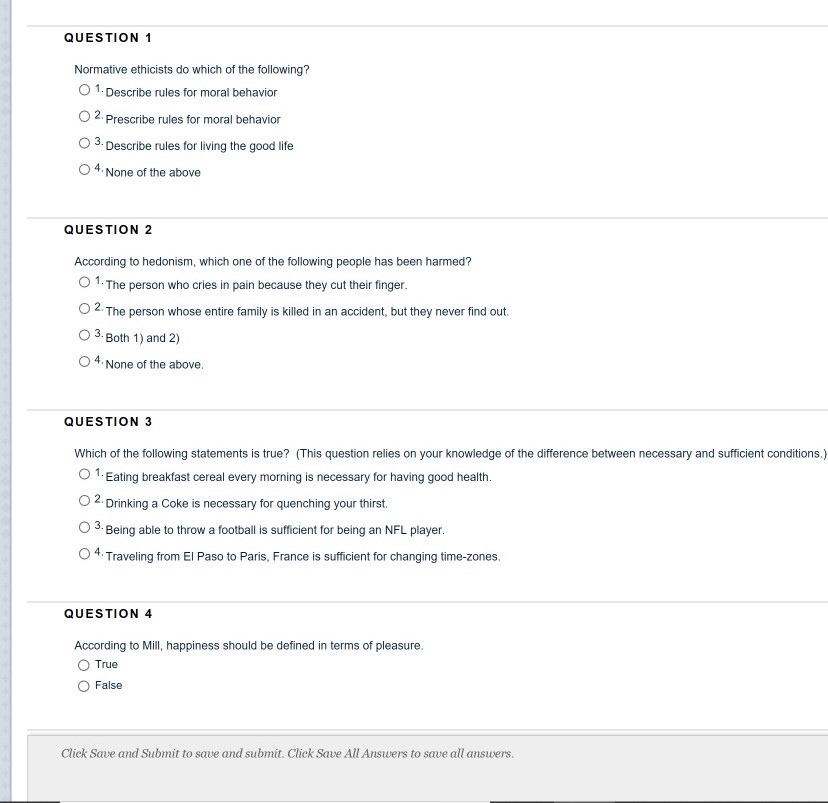This image depicts a digital multiple-choice quiz, likely designed for educational practice or testing purposes. The interface features a series of questions with selectable options. At the very top, the quiz title remains unmentioned, but the questions unfold as follows:

1. **Question 1: "Normative ethicists do which of the following?"**
   - Option 1: Describe rules for moral behavior.
   - Option 2: Prescribe rules for moral behavior.
   - Option 3: Describe rules for living the good life.
   - Option 4: None of the above.

2. **Question 2: "According to hedonism, which of the following people has been harmed?"**
   - Option 1: The person who cries in pain because they cut their finger.
   - Option 2: The person whose entire family is killed in an accident but they never find out.
   - Option 3: Both one and two.
   - Option 4: None of the above.

3. **Question 3: "Which of the following statements is true?"**
   - The question requires the participant to distinguish between necessary and sufficient conditions.

4. **Question 4: "According to MII, happiness should be defined in terms of pleasure."**
   - Answer options: True or False.

Each question progresses with a clear structure, allowing the user to select answers that best fit the given scenarios. The final question deviates from the multiple-choice format, offering a straightforward true or false choice.